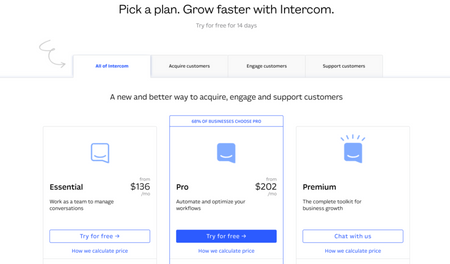The web page presents an organized and visually appealing layout to help users choose the best Intercom plan to accelerate business growth. 

### Header
At the top of the page, in bold black text, the heading reads: "Pick a Plan, Grow Faster with Intercom." 

### Navigation Tabs
On the right-hand side, a gray squiggly line directs attention to a set of tabs. The currently selected tab, "All of Intercom," features a white background with dark blue text. The other unselected tabs, displayed in mid-gray with black text, are labeled: "Acquire Customers," "Engage Customers," and "Support Customers."

### Introduction
Beneath the tabs, bold black text states: "A new and better way to acquire, engage, and support customers."

### Plans
#### Essential Plan
On the left, a light gray-bordered square encloses another blue square featuring a curved line. To the left within this square, the text "Essential" is displayed in black. Above, in small gray text, it reads "From." Beneath, bold black text indicates the price: "$136." Adjacent, regular black text describes: "Work as a team to manage conversations." A clickable button with a white background and blue border, containing blue text reading "Try for Free" and an arrow pointing to the right, invites user engagement.

A note below the rectangle, titled "How We Calculate Price," explains the cost structure. Further blue text highlights, "68% of businesses choose Pro."

#### Pro Plan
A dark blue square with a smiley face line mirrors the previous graphical style. This plan, labeled "Pro," shows a bold price of "$202" below the introductory word "From." The description reads: "Automate and optimize your workflows." A dark blue button with white text, "Try for Free," and an arrow pointing right, encourages immediate action. Another informational rectangle below reads: "How We Calculate Price" in blue text.

#### Premium Plan
The final plan displays a dark blue square with rays emanating from a head, featuring a white mouth and thought bubble. The plan is labeled "Premium" in bold black text, with a description stating: "The complete toolkit for business growth." A dark blue-bordered rectangle contains blue text that reads, "Chat with Us." Below, in hyperlinked blue text, there is another note on pricing: "How We Calculate Price."

This detailed layout provides users with all necessary information to make an informed decision about which Intercom plan best suits their business needs.